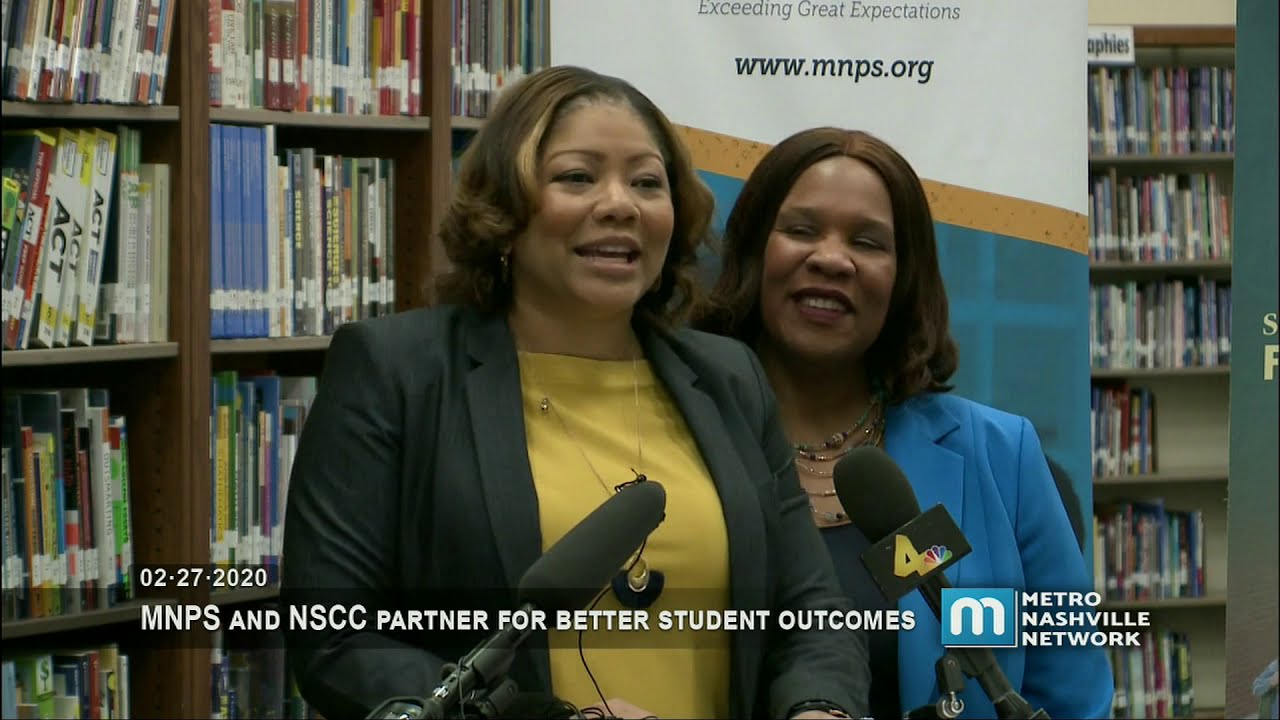In this horizontal rectangular image, we see two African-American women standing centrally in what appears to be a library. They are framed by bookshelves filled with books, some of which are visible to the left and say "ACT" repeatedly, while to the right the bookshelves are slightly blurred out. Behind them is a sign that reads "Exceeding Great Expectations www.MNPS.org."

Both women are smiling and facing forward, each speaking into microphones. One of the microphones prominently displays a gold number 4 with the NBC logo. The woman on the left is wearing a gold t-shirt paired with a black jacket and a thin chain necklace. The woman on the right is dressed in a blue jacket over a black shirt, accessorized with multiple necklaces.

At the bottom left, the date "02-27-2020" is displayed, alongside the text "MNPS and NSCC partner for better student outcomes." In the bottom right corner, there is the Metro Nashville Network logo, featuring a white "M" on a blue background.

The detailed backdrop includes more than just books; there is a wall behind the second woman with a blue design, a brown border, and a white top, adding further context to the setting as a well-organized library space.